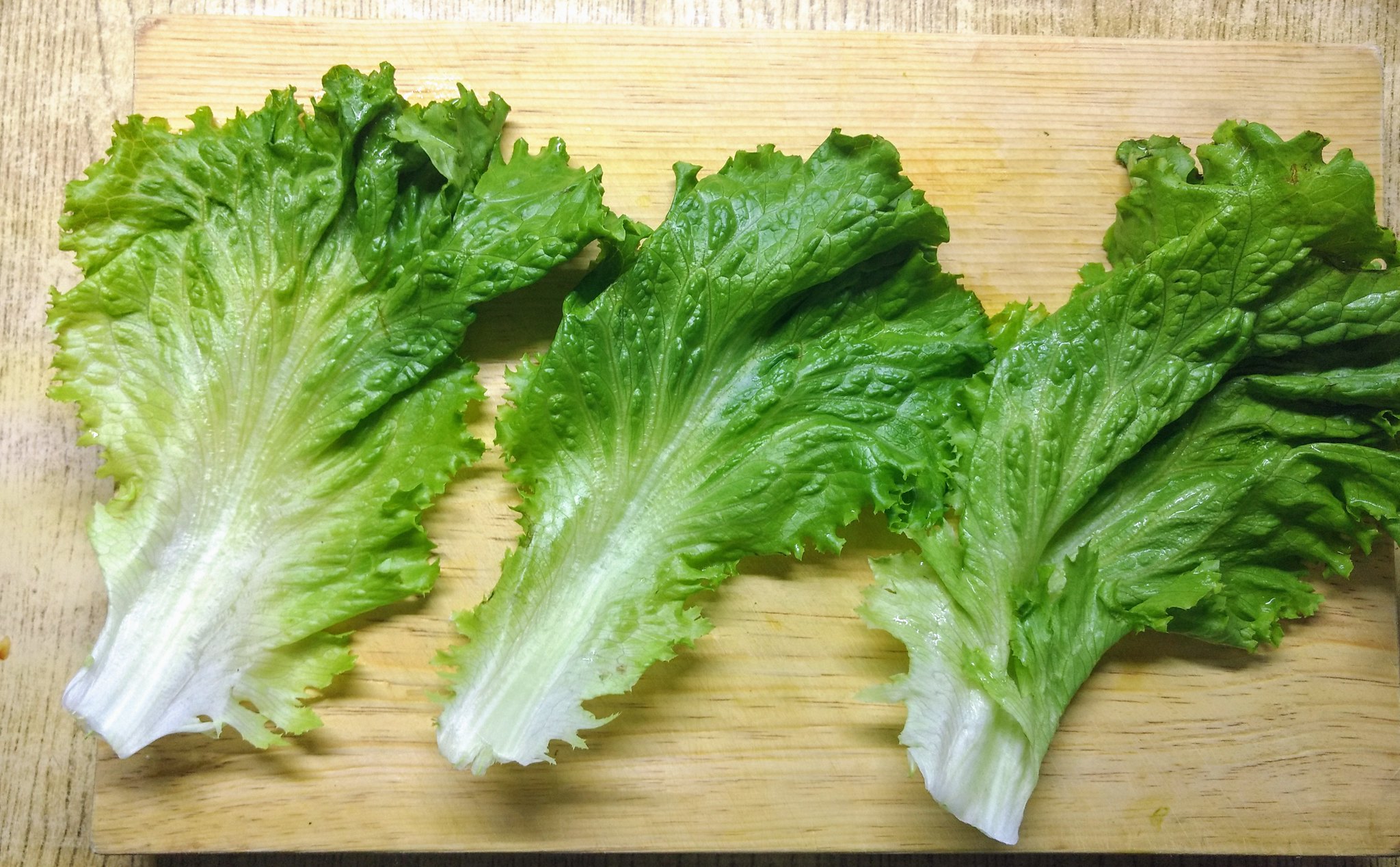This photo showcases three large, healthy, and freshly washed romaine lettuce leaves arranged on a butcher block-style wooden cutting board. The vibrant green leaves, which are similar in size, display a shiny texture, indicating they were recently washed and patted dry. The tops of the leaves are a dark green, gradually transitioning to a much paler green and then white at the thick, sturdy stems. The cutting board, which features a light brown color with darker brown lines, rests on a wooden table that matches closely in color and pattern, creating a cohesive and earthy backdrop for the fresh produce.